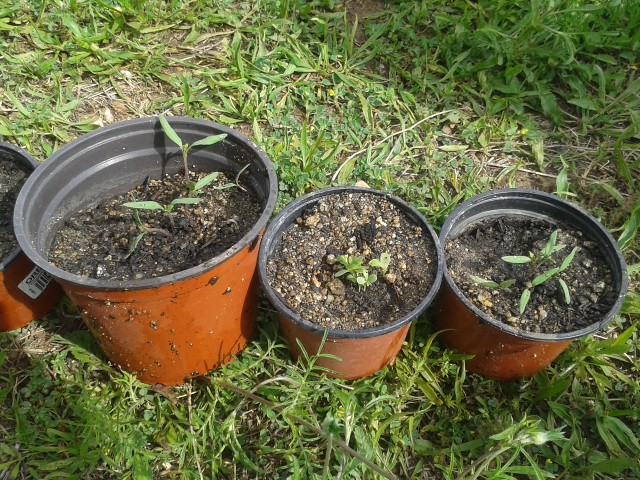The image showcases a grassy outdoor setting featuring four pots arranged in a row. The grass forms a lush, solid green backdrop typical of spring, with some dirt peeking through near the top. The pots are predominantly orange on the exterior and black on the interior, though the leftmost pot is only partially visible with a white sticker on its side. The visible portions reveal that the pots are plastic, filled with dark soil that has white spots and rocks mixed in.

In the second pot, fully visible, a young plant emerges, characterized by a single stick with two small green leaves. Similarly, the third pot also supports young plants, each sprouting leaves. The fourth pot, although partially cut off and slightly larger than the others, also reveals budding growth with a cluster of small green leaves.